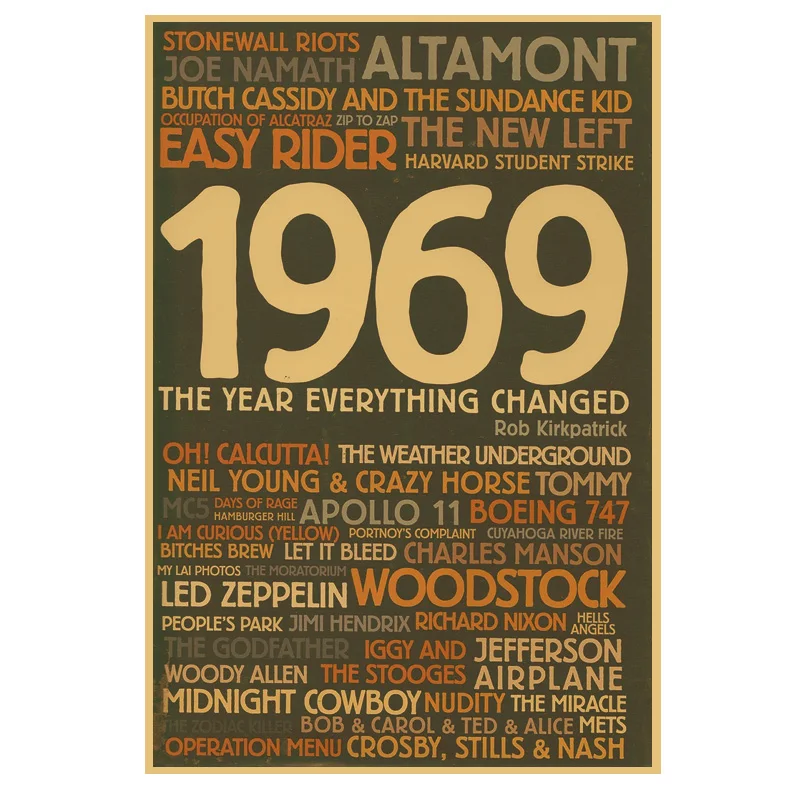The poster has a dark gray background with a beige outline and prominently displays the large, bold numbers "1969" in the upper middle. Below the numbers, in tan and yellow colors, the text, "The Year Everything Changed," is written. The top part of the poster features alternating orange, gray, and yellow text listing significant events and names, such as "Stonewall Riots," "Joe Namath," "Butch Cassidy and the Sundance Kid," "Occupation of Alcatraz," "Zip to Zap," "Easy Rider," "The New Left," "Harvard Student Strike," and "Altamont." Toward the bottom half, additional events and figures are listed, including "Oh! Calcutta," "The Weather Underground," "Neil Young and Crazy Horse," "Tommy," "MC5," "Days of Rage," "Hamburger Hill," "Apollo 11," "Boeing 747," "I Am Curious (Yellow)," "Bitches Brew," "Let It Bleed," "Charles Manson," "Woodstock," "Richard Nixon," "The Stooges," "Midnight Cowboy," and "Crosby, Stills and Nash," among others. The names "Rob Kirkpatrick" and various music and cultural references like "The Stooges," "Jefferson Airplane," and "Jimi Hendrix" are also interspersed throughout the poster.